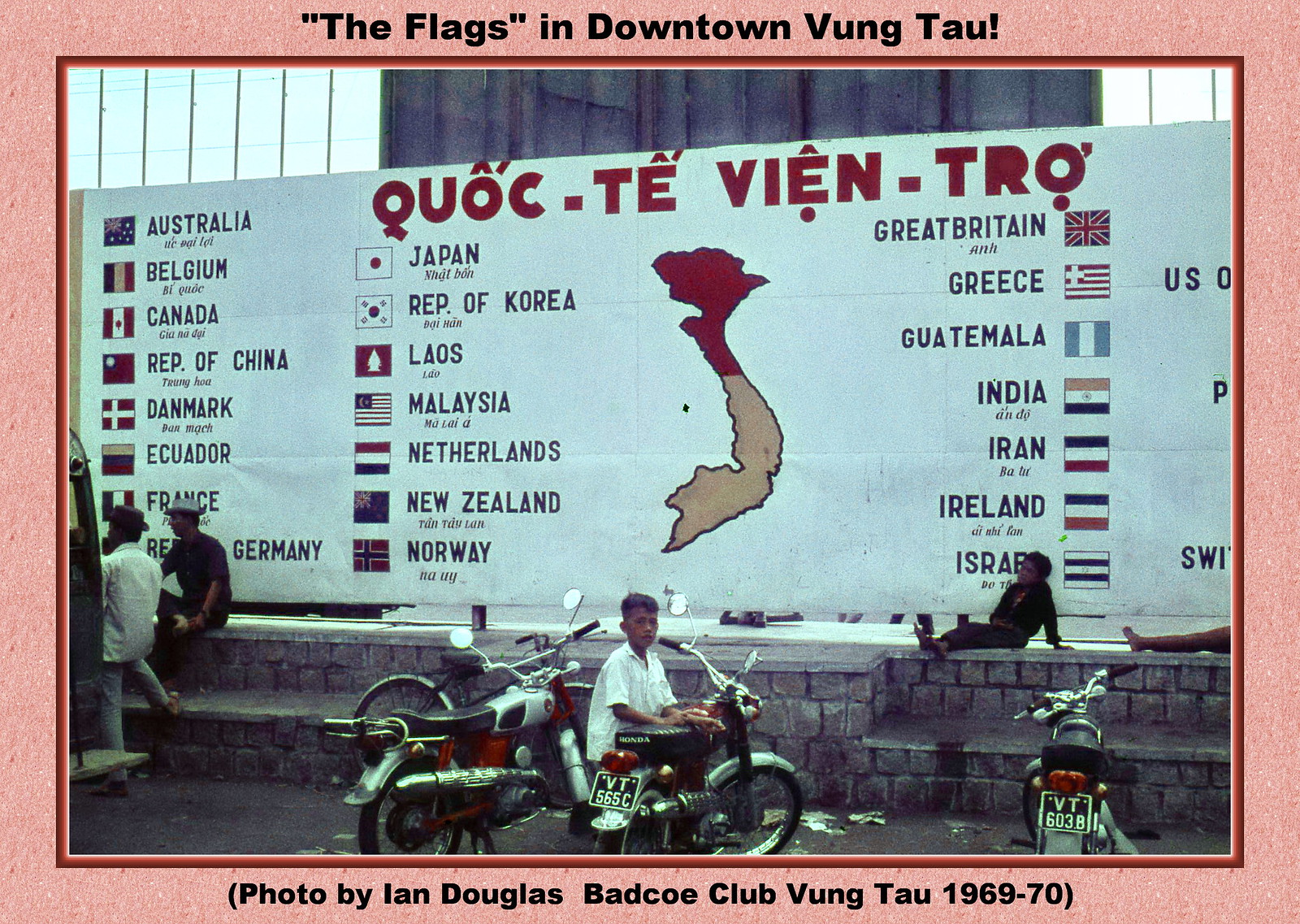This photograph, dated from 1969 to 1970, captures a vibrant scene in downtown Vung Tau, a city in Vietnam. The image prominently features a large white banner adorned with red Vietnamese text at the top, proclaiming "Quoc Te Vientreau" and subtitled "The flags in downtown Vung Tau." The banner showcases flags from numerous countries, including but not limited to Australia, Belgium, Canada, Republic of China, Denmark, Ecuador, France, Germany, and Japan, with a map of Vietnam centrally displayed. This suggests the international presence and involvement in Vietnam during the war era.

The foreground of the photograph is bustling with activity; several people are perched on a brick wall or stone platform in front of the banner. Among them, a young man stands out as he looks back at the photographer, gripping the handlebar of a motorbike. Additional motorbikes flank him, one to his left and another to his right. The scene is illuminated by daylight, indicating that the photograph was taken outdoors during daytime, capturing a historical moment brimming with life and international significance. The photo credits Ian Douglas and notes the Batco Club Vung Tau as a part of this archival glimpse into the past.